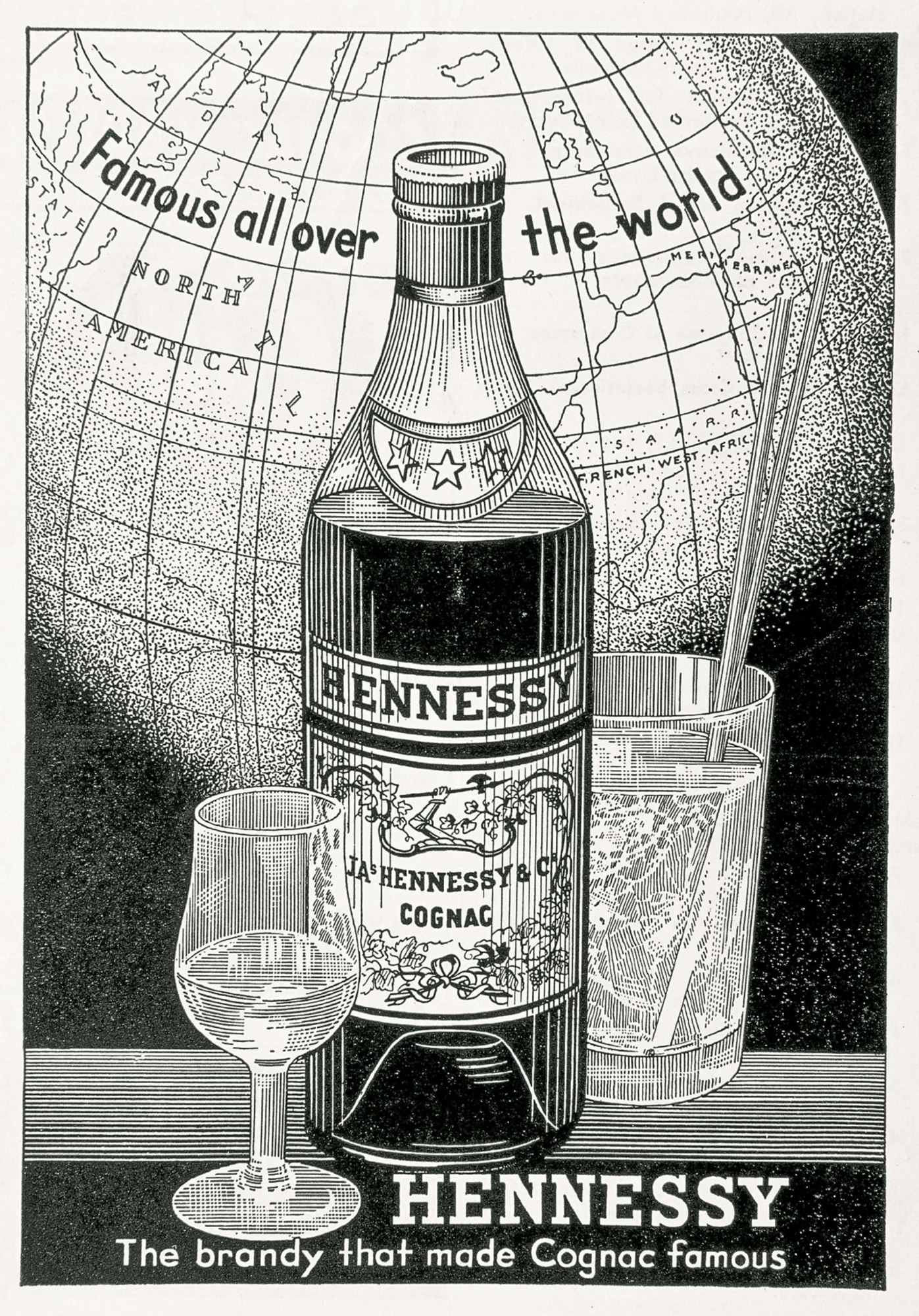This vintage-style black and white advertisement for Hennessy cognac features a stenciled illustration with an intricate design composed of lines and dots. Front and center is a prominently labeled bottle of Hennessy, imprinted with "J.A. Hennessy & Co." and "Cognac." The bottle is unopened and full, suggesting a premium, untouched product. To the left of the bottle is a partially filled wine-shaped whiskey glass, while to the right, behind the bottle, is a nearly full traditional mixed drink glass with two straws. The backdrop of the scene is a rectangular depiction of a globe, shaded meticulously with dots, showcasing continents including North America. Boldly inscribed across the globe is the phrase "Famous all over the world." The composition is capped with the slogan at the bottom, "Hennessy, the brandy that made Cognac famous," emphasizing the global recognition and historical prestige of the Hennessy brand.